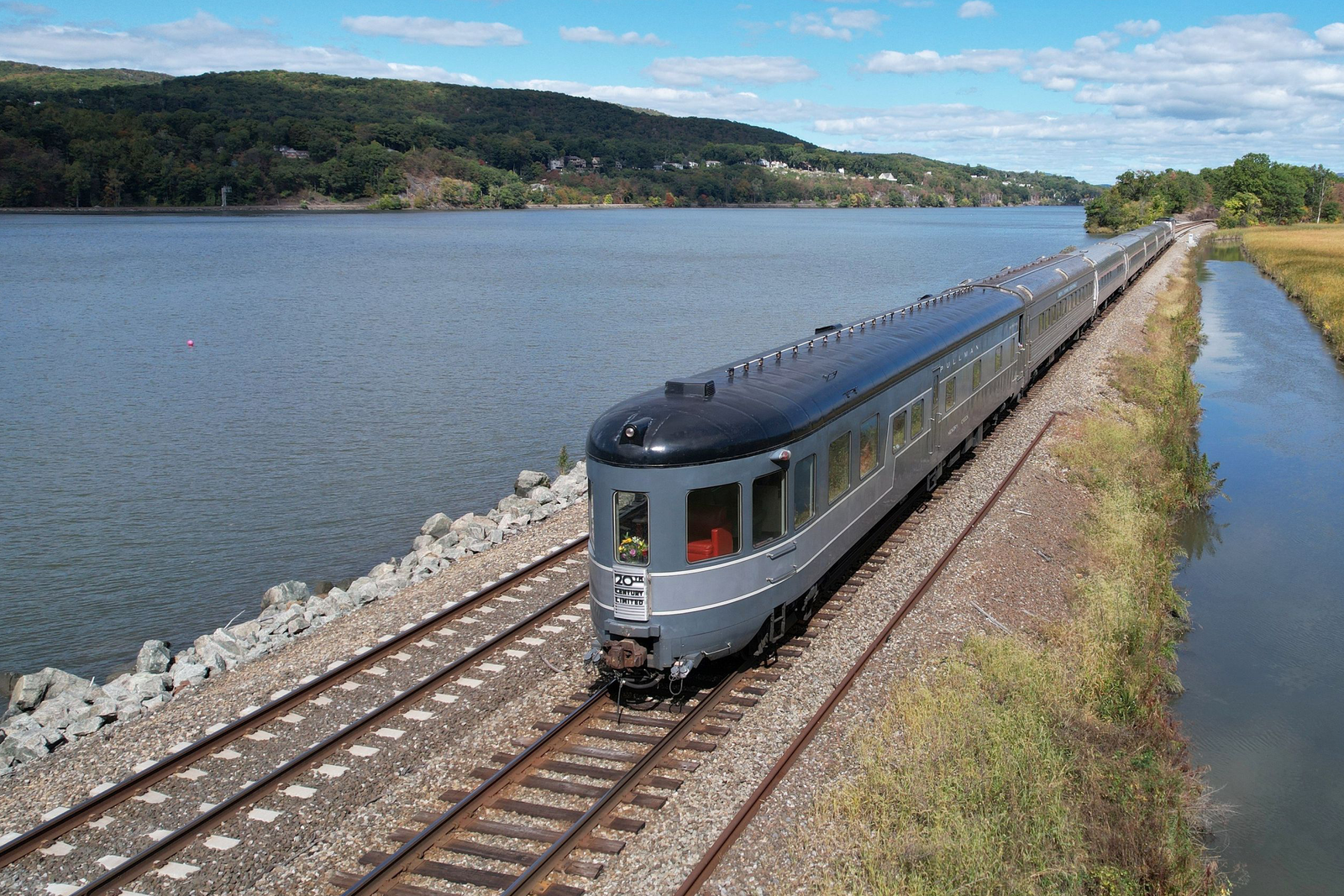In this aerial photograph, a silver commuter train is seen in motion, captured in sharp detail at the front and slightly blurred at the rear, suggesting its high speed. The train is traveling on dual tracks laid on a narrow, elevated embankment that splits a calm, blue body of water, likely a river or lake. The water dominates the scene, especially on the left side of the tracks, while a grassy, rocky terrain with sparse scrub brush edges the right. Behind the train, on the left, a larger expanse of water gradually tapers off to the right, giving way to a verdant hilly area in the background. A small town can be discerned nestled within this green landscape, close to the frosty water's edge. The backdrop features distant mountains under a picturesque blue sky dotted with white clouds, completing the tranquil yet dynamic scenery.